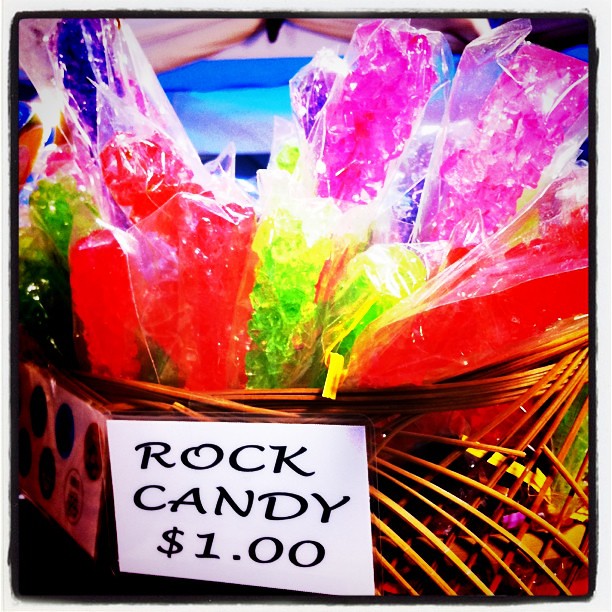The image depicts a light brown wicker basket filled with an assortment of colorful rock candy, each piece wrapped in plastic. The vivid colors of the rock candy include shades of pink, green, red, blue, purple, and indigo, resembling clusters of gems. Attached to the front of the basket is a small, square, white sign with black text that reads, "Rock Candy $1." The background of the image hints at a blue structure, potentially another basket, and a fabric or accent piece draped overhead, suggesting the setting might be within a tent or market stall. The entire scene is bordered by a white edge, giving the impression that this is a printed photograph.